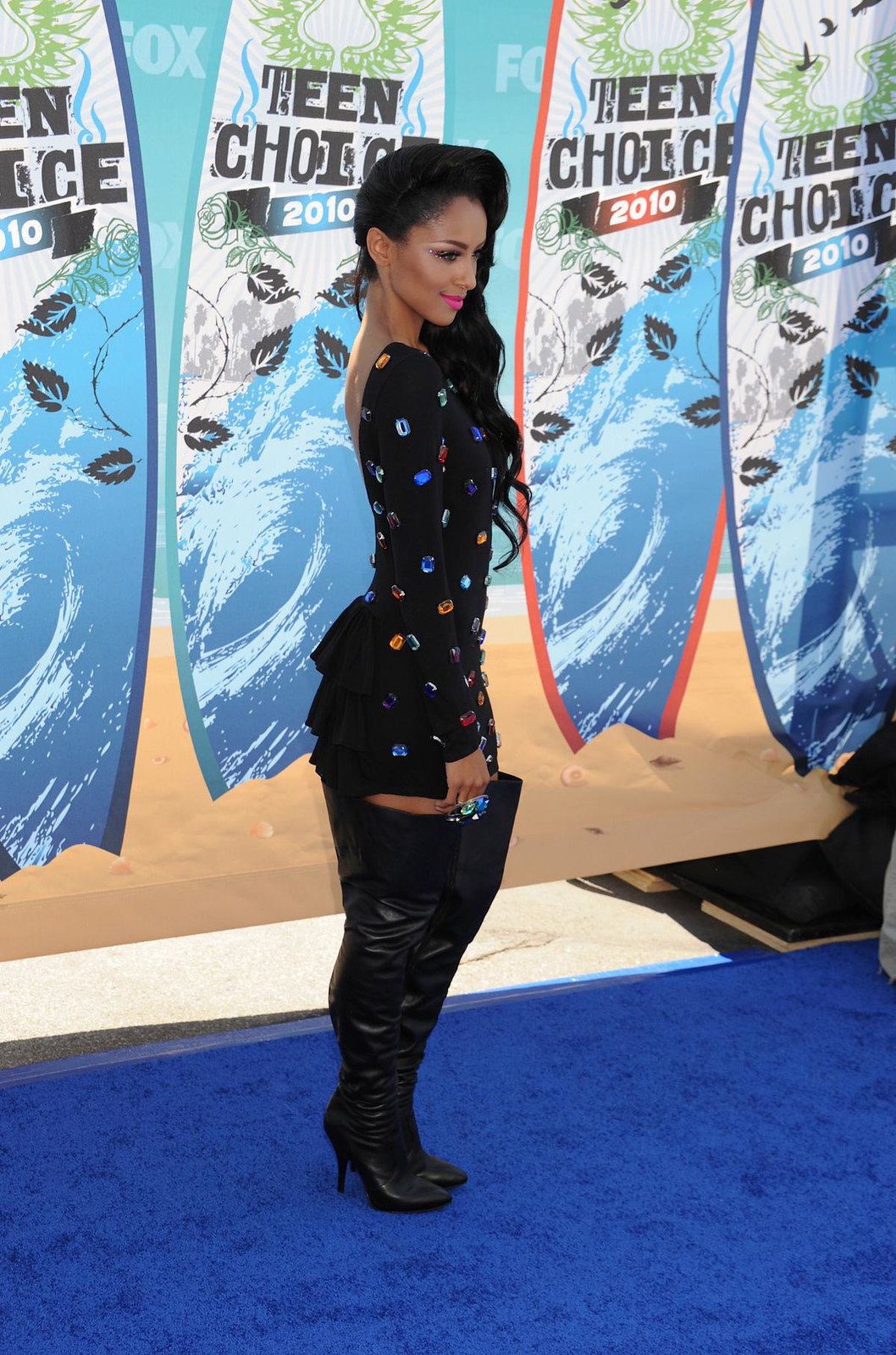In this vertically aligned rectangular photo, a glamorous woman is captured from a side view while standing on a blue carpet, possibly at the Teen Choice Awards 2010. She is dressed in a very short, tight black dress adorned with large encrusted jewels and colorful specks. Her outfit is complemented by thigh-high black leather boots with heels. The woman, who has dark, long wavy hair pulled over her left shoulder, is smiling and wearing pink lipstick. She also sports chunky rings that add to her glamorous look. Behind her, four surfboard-shaped banners hang, displaying "TEEN CHOICE 2010" in black letters, with variations in the year’s color scheme—three in blue and one in red, all with a white background. The banners feature a water effect with leaves and are sponsored by Fox TV. The setup suggests that she is attending or modeling at the event, with the scene appearing to be outside, despite some indication of a secondary brown flooring behind the banners.